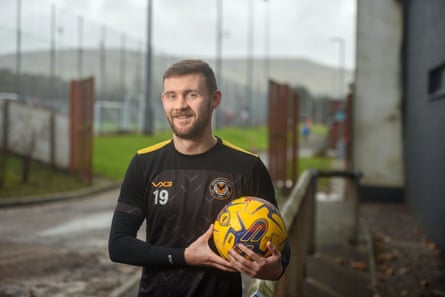The photograph features a smiling, bearded man standing outdoors, holding a yellow and blue soccer ball to his left. He is dressed in a black long-sleeved jersey adorned with yellow stripes on the shoulders and the number 19 in white letters on the right side of his chest. The man, who has short brown hair and a close-cropped mustache and beard, is captured from head to waist against a blurry background. This background reveals a soccer field bordered by tall wire fences, a concrete wall on the right, and a road on the left. The weather appears gray, casting a muted sheen over the image. The bright yellow soccer ball he holds features geometric blue patterns, contrasting with the dim ambiance of the scene.